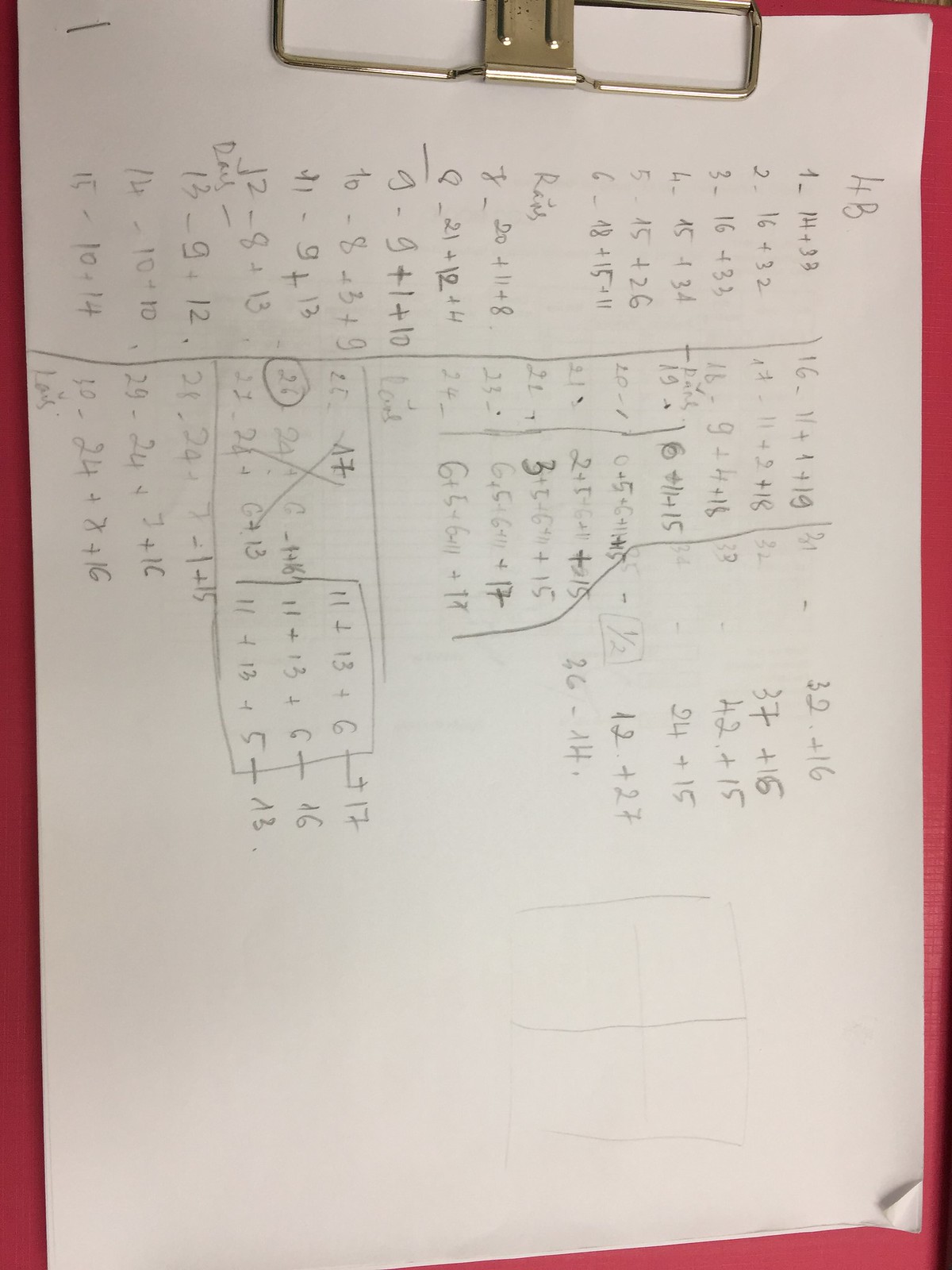A detailed photo captures a student diligently working through a mathematical assignment on a white piece of paper secured to a vibrant red clipboard. The paper, devoid of any grid lines, is filled with a series of arithmetic problems, methodically listed from numbers 1 to 12. The math problems, such as 14 + 33, 16 + 32, 16 + 33, and 16 + 45, span the length of the page, reflecting the student's meticulous efforts. A small folded edge is visible on the bottom right-hand corner of the paper, subtly disrupting the otherwise smooth surface. Nearby, a faintly drawn pencil square can be discerned, adding a touch of personalization to the homework.